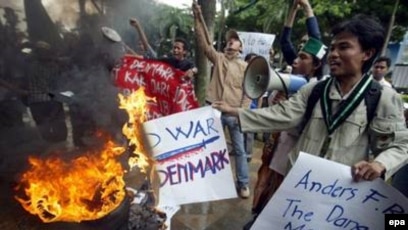In the photograph, a vivid scene of an outdoor protest unfolds, characterized by striking elements that capture the intensity and fervor of the moment. Centered in the image is a man wearing khaki-colored clothing and a strap around his neck that could be a press pass. He is clasping a partially burned, handwritten sign that reads "war" and "Denmark," adorned with a crude drawing of a sword. The sign is being held over a flaming trash can or barrel, which emits thick, black smoke that adds to the chaotic atmosphere. In his other hand, the man holds another sign with the partially visible text "Anders F..." while surrounding him are additional protesters, some of whom brandish megaphones and hold aloft various banners.

The scene is further animated by another protester, distinguishable by a green hat, who is vocally advocating for their cause through a bullhorn. A red sign and two men with their arms raised—one in a tan shirt and the other in an off-white shirt—add to the dynamic composition. The background reveals a verdant, heavily wooded area, hinting at a setting possibly in South America, despite the mention of Denmark on the burning signs. Amidst the protesters, a black box labeled "EPA" in white text can be seen in the bottom right corner, suggesting the image might be a screenshot from a video. The overall atmosphere is charged, with people evidently dressed for warm weather, adding to the palpable tension of this powerful protest scene.